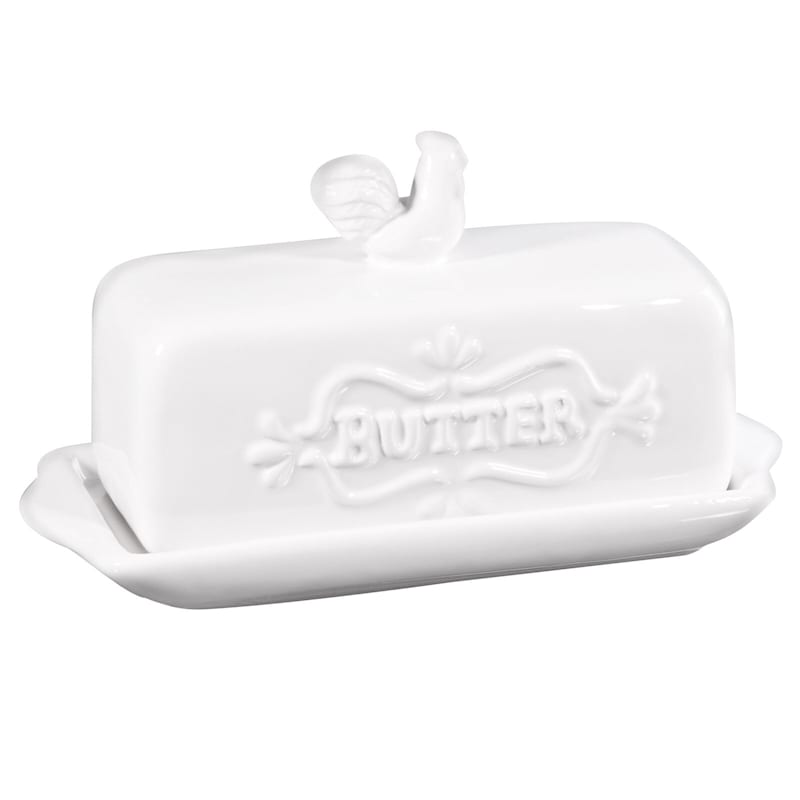The image features an all-white, retro-style butter dish set against a matching white background. The dish comprises a rectangular tray with slight protrusions on the ends for easy handling, designed to hold a stick of butter. The domed lid, also white and slightly rounded, fits seamlessly over the tray. The word "butter" is prominently centered and inscribed on the side of the lid, accented by a decorative, candy-wrapper-like border with petal elements. At the very top of the lid, there is a small rooster figure serving as a handle for lifting the lid, enhancing its farmhouse charm. The entire dish has a shiny, creamy white finish.